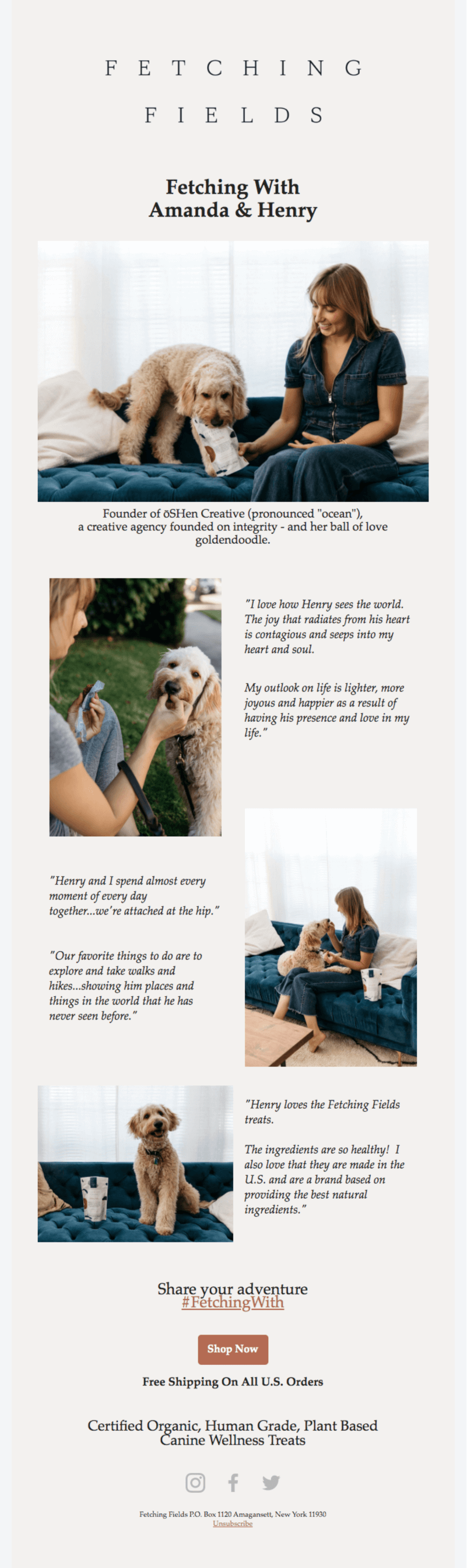The webpage features a light gray background with "FETCHING FIELDS" prominently displayed in black capital letters at the top. Directly below, the header reads "Fetching with Amanda and Henry." Centered on the page, there is an image of a tan-colored dog sniffing a bag of treats, next to a person with long brown hair, pale skin, wearing a blue top and blue pants, who is sitting on a blue button-tufted couch and holding the bag of treats.

Further down on the left, there is a smaller thumbnail image of a woman kneeling in the grass, wearing a blue short-sleeved shirt and blue jeans. She has pale skin and is feeding a treat to a white long-haired dog.

To the right of this thumbnail, there are two small paragraphs of text that are unreadable due to their size. Below, on the left-hand side, more text is visible but also too small to be read. Adjacent to this text block is another picture: the same person from the main image, this time interacting with the tan-colored dog, which has its front paws on her lap. The person’s face is partially obscured by her brown hair as she feeds the dog a treat.

Continuing down the page, there is a small image of the tan dog sitting on the blue button-tufted couch, looking forward. To the left of the dog is a bag of animal treats. To the right of this image, more text appears but remains too small to decipher.

The bottom section of the webpage features the phrase "Share your adventure" in black letters, followed by the hashtag "#FetchingWith." Below this, there is an orange button with text that is too small to be read.